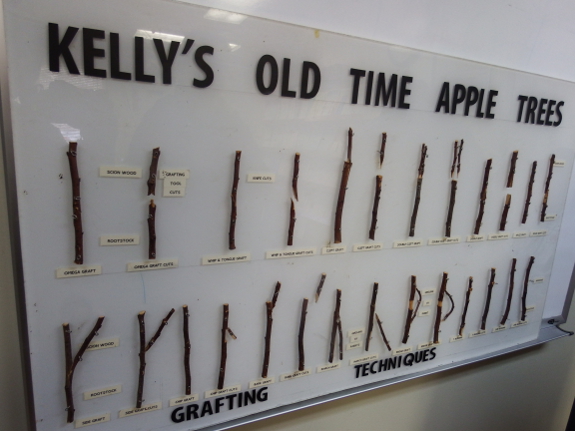The image displays an educational poster titled "Kelly's Old Time Apple Trees," mounted on a white marker board and leaning against it. The poster features two rows of multiple brown apple tree sticks, each carefully labeled on cream-colored paper. The text at the top reads "Kelly's Old Time Apple Trees" in all capital letters, while at the bottom, the text "Grafting Techniques" highlights the main focus of the display. The sticks between these lines demonstrate various grafting methods, showcasing at least 28 different techniques to fuse apple tree stems for crossbreeding different apple varieties. Each method is illustrated with real samples of apple tree grafts, labeled meticulously to detail the different ways to cut and tie the stems. Additional small writings on the cream-colored labels provide further information about each grafting technique. The entire setup is on a white wall, making the educational content striking and accessible.